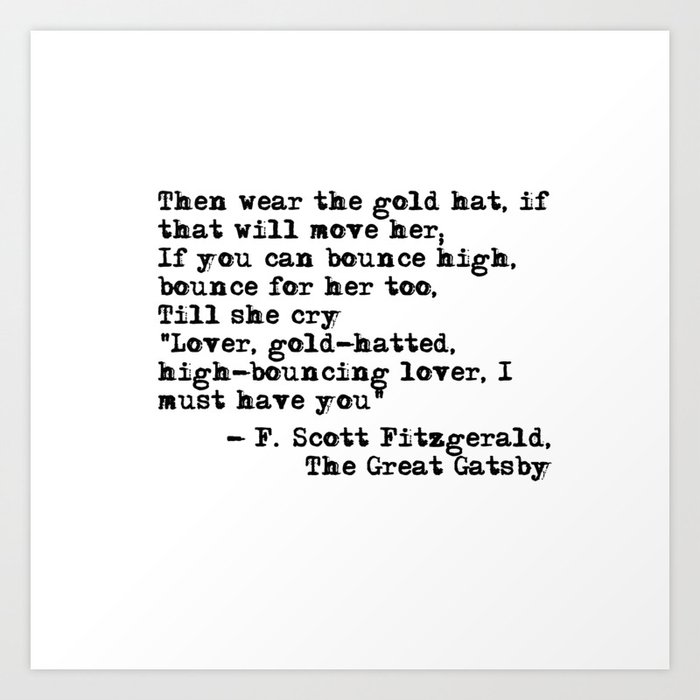This image features a neatly trimmed square with a cream border surrounding a white background. In the center, there is a typewritten quote in a black sans-serif font, characteristic of a typewriter's imperfect ink distribution, giving some letters a slight double imprint. The text reads:

"Then wear the gold hat, if that will move her; if you can bounce high, bounce for her too, till she cry 'Lover, gold-hatted, high-bouncing lover, I must have you.'" 

This passage, attributed with a dash to F. Scott Fitzgerald, originates from his novel "The Great Gatsby." There is nothing else in the image, making the text the focal point, emphasized by its potential utility for social media posts or literary discussions.